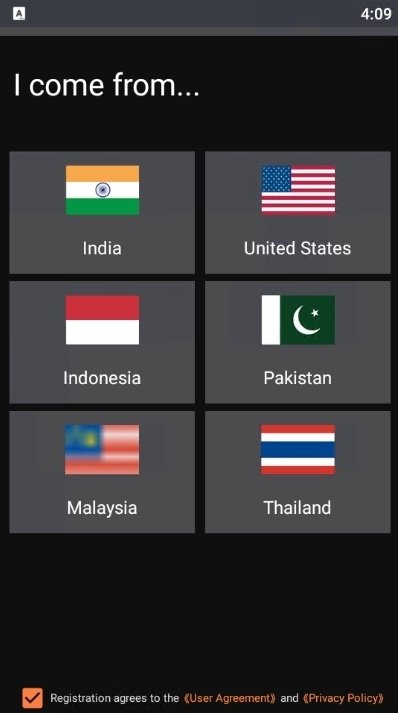The image features a stark black background with various elements and text. At the top center, a white rectangular box contains a gray letter "A" on the left, and on the right, the digital time displays "4:09".

Below, against the black background, the text reads, "I come from...". This is followed by six distinct gray rectangles, each representing a country with its respective flag and name. 

1. **India**: The box features the Indian flag above the text, with horizontal stripes of orange, white, and green.

2. **United States**: This rectangle displays the American flag with its characteristic red and white stripes and a blue field adorned with 50 white stars.

3. **Indonesia**: The Indonesian flag is depicted with a horizontal red stripe above a white stripe.

4. **Pakistan**: The Pakistan flag has a green field with a white vertical stripe on the left, featuring a white crescent and star.

5. **Malaysia**: The Malaysian flag is noticeably blurred, but it seems to display colors including yellow, blue, red, and white.

6. **Thailand**: The flag of Thailand has horizontal stripes of red, white, blue, then white, and red again.

At the bottom of the image is an orange box featuring a black checkmark. The text inside this box reads, "Registration agrees to the," followed by "an armistice agreement". Below, in parentheses and orange text, it states "(private policy)".